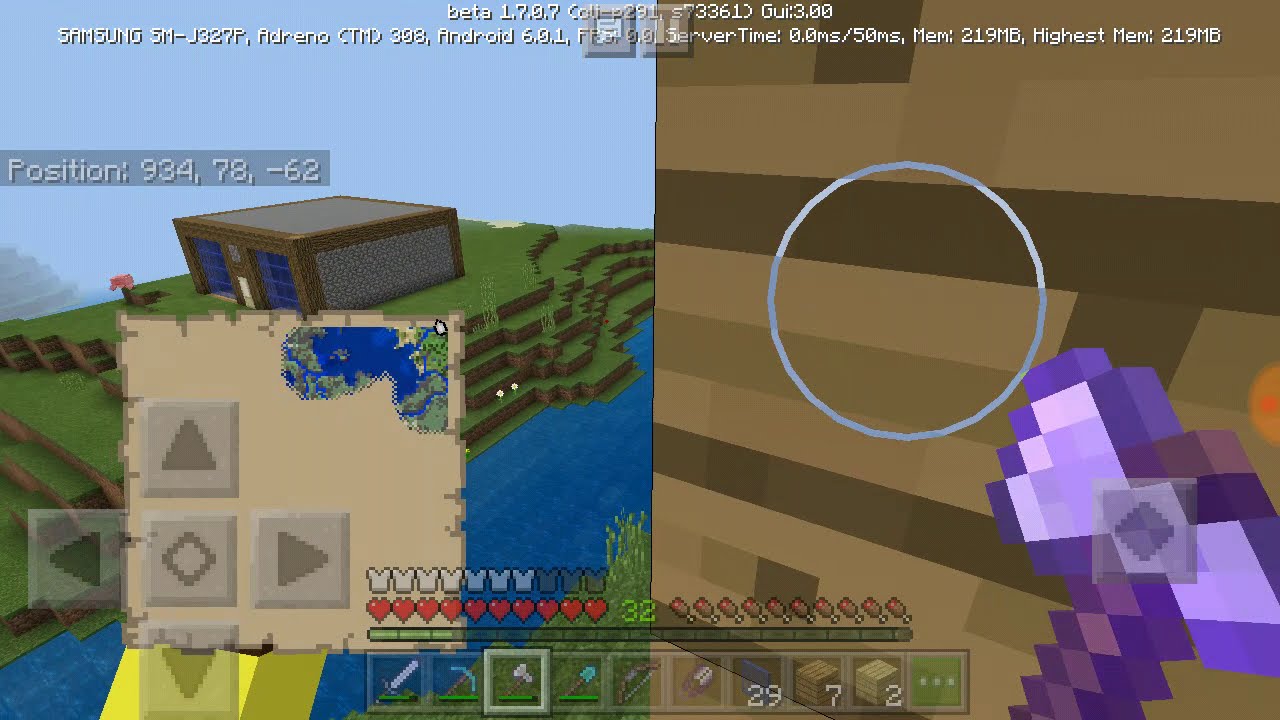The image is a screen capture from a video game, showcasing a split-screen layout. On the left side, there is a highly pixelated map central to the composition, overlayed with directional arrows (up, down, left, and right) and a diamond icon. The map has a predominantly brown color scheme, indicating sand or dirt, with a small body of water in the upper right, bordered by tree lines and adjacent to a terraced grassy plateau with a one-story structure resembling a garage with two bay doors and blue windows. On the right side, the game is depicted in a first-person perspective featuring a pixelated scene reminiscent of an 8-bit style, likely from a game like Minecraft. A purple hammer or object is visible in the character's right hand. The background displays a varied landscape with brown, gray, green, and blue hues, showing a river flowing near the base of a hill topped with the aforementioned structure. Numerical coordinates (94, 78, -62) appear above the building, and standard in-game interface elements, such as weapon choices and life indicators, are present at the bottom of this panel.